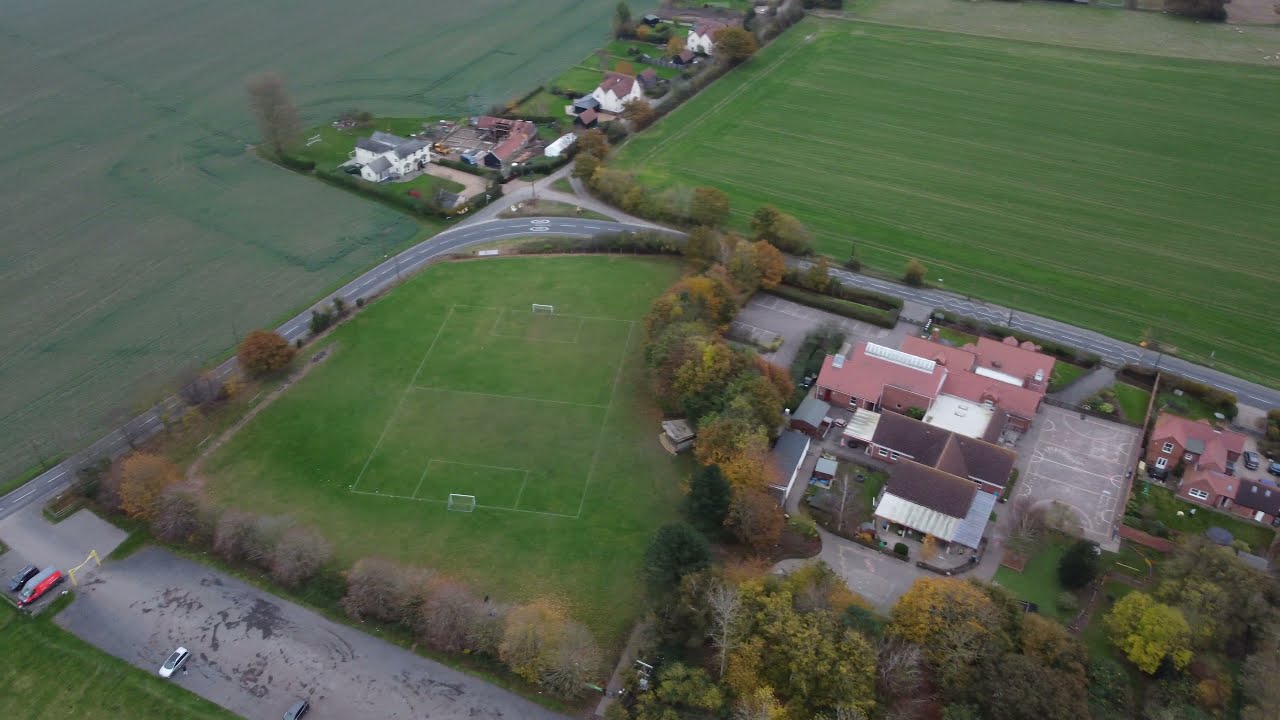This detailed aerial photograph captures a vibrant landscape with a blend of structured and natural areas. Dominating the center-left portion of the image is a soccer field, marked with distinct white lines and equipped with white goals. Surrounding this field are expanses of farmland, contributing to the image's rural charm. On the right bottom part, there's a large building, possibly a school, with a yard that features lines resembling basketball or tennis courts. Adjacent to this are several buildings that include a sizable, two-story, reddish-brown house with A-frame roofs, surrounded by trees and a fence. 

In the upper center of the photograph, a neighborhood unfolds, characterized by white houses with similar reddish-brown A-frame roofs, nestled within green open spaces. A street wraps around the school area, adding a structured flow to the scene. At the back of the photo, both on the right and left sides, expansive green fields stretch out, reflecting the spacious countryside. In the foreground, a parking lot with yellow metal posts is partially occupied by a few cars, enhancing the image's overall impression of an active, well-used community setting. This neighborhood, with its harmonious blend of residential, educational, and recreational spaces, looks picturesque and inviting.